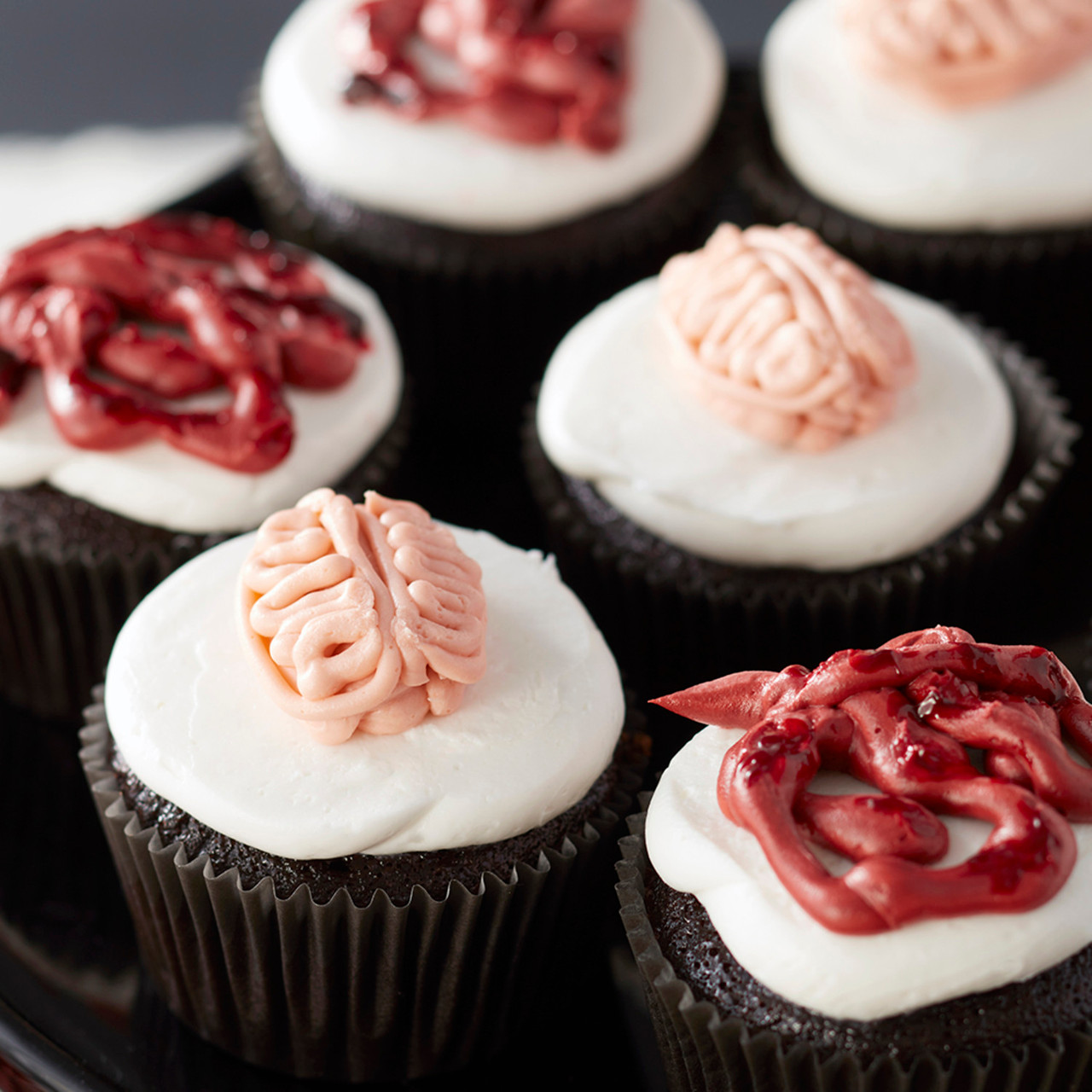This rectangular image, slightly taller than wide, showcases six chocolate cupcakes arranged diagonally from the top-right corner to the bottom-left. Each cupcake, encased in a dark brown, almost black paper wrapper that matches the deep chocolate hue of the cake, is topped with a smooth layer of white frosting. The cupcakes are distinguished by two different decorative patterns on top of the white icing: 

Three cupcakes, distributed in a diagonal line across the middle of the image, feature intricate, brain-shaped designs made from light pink frosting. The remaining three cupcakes, located at the far right and upper left corners, are adorned with a jumbled mess of reddish-brown icing, resembling a random, messy squiggle. The focus of the camera highlights the two cupcakes at the front, gradually blurring towards the back, giving prominence to the detailed frosting work. A subtle, gray and white background peeks through the top left corner, enhancing the overall composition.